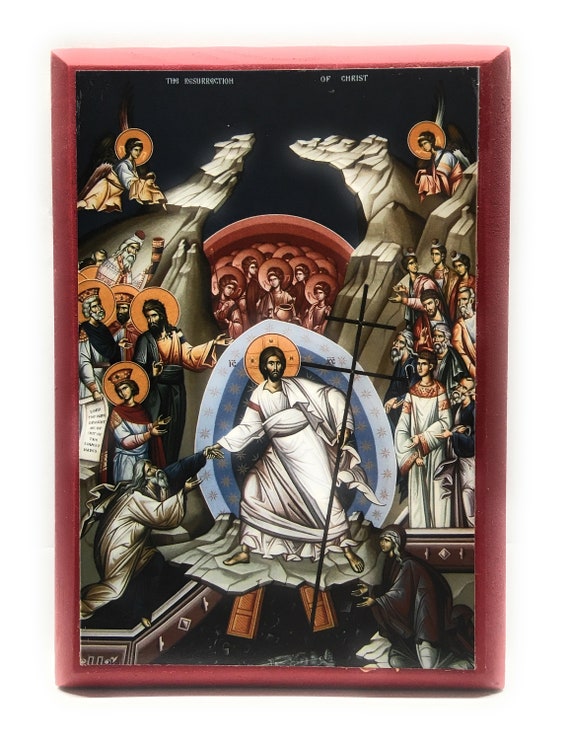The image is a full-page color illustration titled "The Resurrection of Christ," prominently displayed in small white font at the top. At its center is a figure of Jesus Christ, adorned in a white robe and illuminated by a golden halo. He stands, seemingly floating, surrounded by a diverse group of people. To the left, figures that resemble apostles can be seen, while on the right, characters don medieval-looking attire. Above Christ, a gathering of reddish angels, each marked by a circle behind their heads, adds a divine layer to the scene. The background is deep blue, contrasted by light gray or brown mountainous terrain, giving the depiction a sense of depth and atmosphere. The entire composition bears a visual style that harkens back to Greek Orthodox iconography, though it appears more modern and less traditional. The illustration captures a moment of reverence and celestial wonder, as all the surrounding figures gaze intently at Christ.